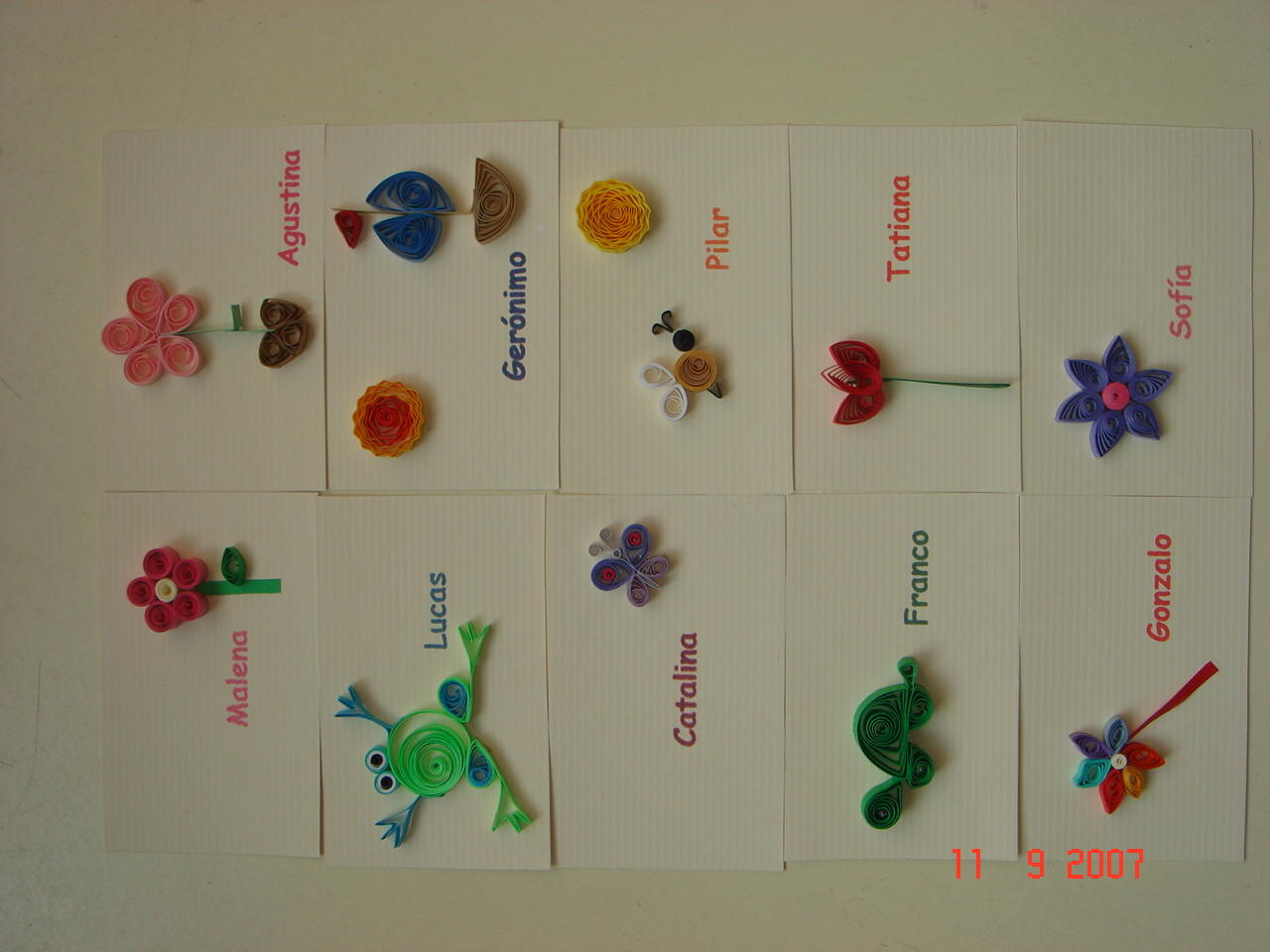The image, taken on 11-9-2007, shows ten name cards arranged on a dull gray background under dim lighting. The photo is rotated to the left. Each card, which appears to be about 3x5 in size, has a child's name written in colored markers — darker colors for boys and lighter, such as pink, for girls. The cards are adorned with raised plastic decorations featuring cheerful and juvenile designs of animals and flowers.

From left to right, starting at the bottom, the names and decorations are as follows:
1. Melina with a pink flower.
2. Augustina with a pink flower.
3. Lucas with a green and blue frog.
4. Geronimo with a little sun and a design that could be a flower or a boat.
5. Catalina with a small butterfly.
6. Pilar with a bumblebee and a sun.
7. Franco with a green turtle.
8. Tatiana with a red flower.
9. Gonzalo with a multicolored flower.
10. Sofia with a purple and pink flower.

The cards are arranged in two rows of five each, creating a bright and cheery display despite the dimly lit setting.